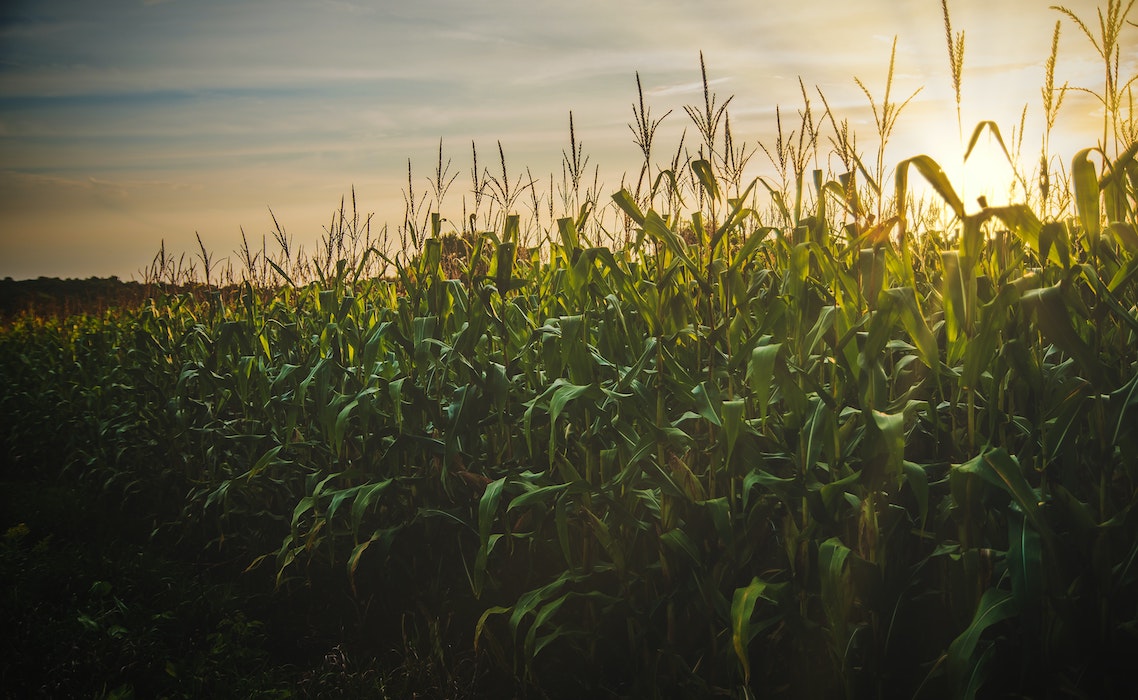A stunning photograph captures an expansive cornfield stretching out towards the horizon. The lush green leaves of the corn plants droop slightly, indicating they are thriving under a well-maintained irrigation system and optimal sunlight. Dominating the sky above, clusters of clouds float with patches of blue peeking through, creating a dynamic backdrop. In the top right corner, the sun shines brightly with a striking yellow hue, casting a warm glow across the landscape. The field, punctuated by tall stalks of mature corn, suggests this area is likely a significant contributor to the country's abundant corn crop. In the left background, gentle hills rise against the sky, adding depth to the scene. The interplay of light and shadows with the sun's rays illuminating the field and creating darker green and almost blackish tones in the lower corners adds a dramatic effect, emphasizing the beauty and productivity of this vibrant agricultural landscape.